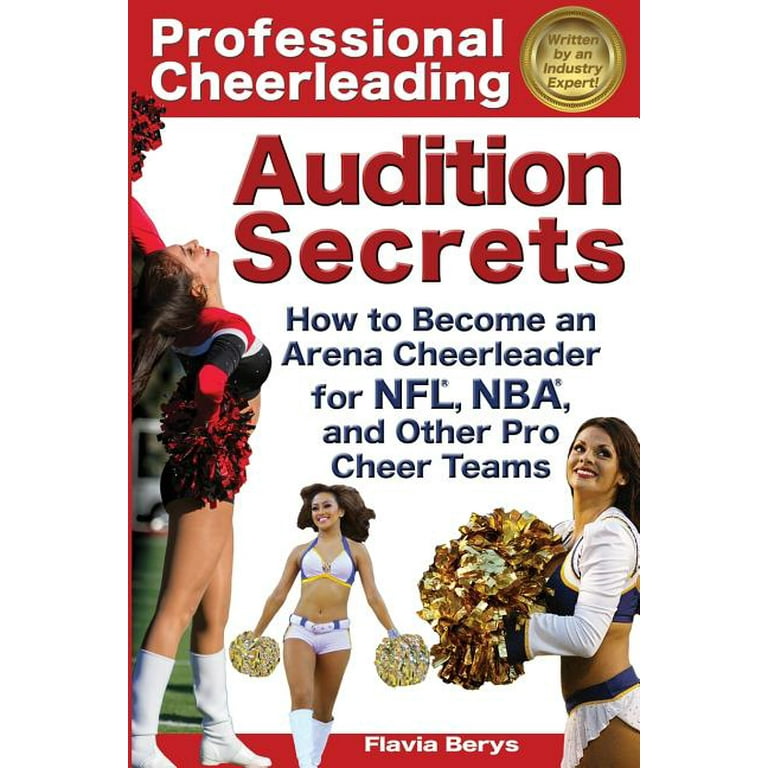This detailed cover of the book "Professional Cheerleading Audition Secrets" prominently features a well-organized layout with distinct text and images. Across the top, a red horizontal strip displays the title "Professional Cheerleading" in white text. Adjacent to this, a gold circular emblem states, "written by an industry expert!" Below this, the background is predominantly white, with bold red text reading "Audition Secrets" and blue text outlining the subtitle: "How to Become an Arena Cheerleader for NFL, NBA, and Other Pro Cheer Teams."

The central section includes three cheerleader images: 
- On the left, a cheerleader in a black and red outfit, holding matching pom-poms, is striking a dynamic pose.
- The middle cheerleader, dressed in white short shorts and a white bikini top, holds yellow and blue pom-poms.
- The cheerleader on the right wears a blue and yellow top over a long sleeve white shirt, complemented by a white skirt and gold pom-poms.

The layout concludes with another red horizontal strip at the bottom, featuring the author's name "Flavia Berys" in white text. This cohesive design ensures clear communication of the book's purpose and credentials through its structured and vibrant visual elements.